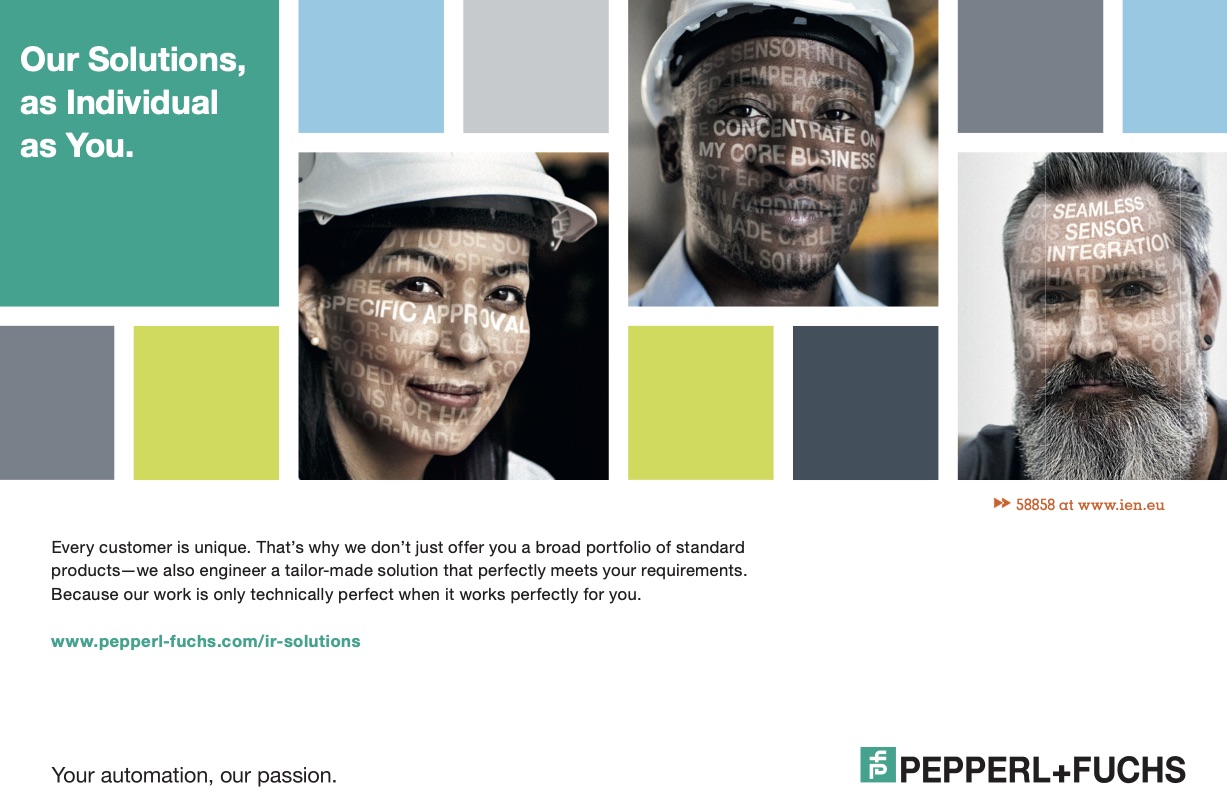Screenshot of a German website focused on customized engineering solutions. The main text reads, "Every customer is unique, that's why we don't offer you a broad portfolio of standard products. We engineer a tailor-made solution to perfectly meet your requirements because our work is only technically perfect when it works perfectly for you."

Displayed prominently is the web address in green text: "www.peperifux.com/IR-solutions." The tagline in green lettering on a white background states: "Automation, our passion by Pepperoi."

Below the tagline, there is another message in white text on a green background: "Our solutions as individual as you."

The layout features multiple colored squares: a gray and yellow square below, with a blue and gray square above a photograph of an Asian woman wearing a white hard hat. The squares have words such as "approval" and "concentration" overlaid on the image. Adjacent to this, there is an image of a black man in a hard hat, accompanied by yellow and black squares. Additionally, there is an image of an older man with a large, grayed-out beard, framed by gray and blue squares. 

The website appears to advertise bespoke engineered solutions, tailored specifically to each customer's unique requirements.